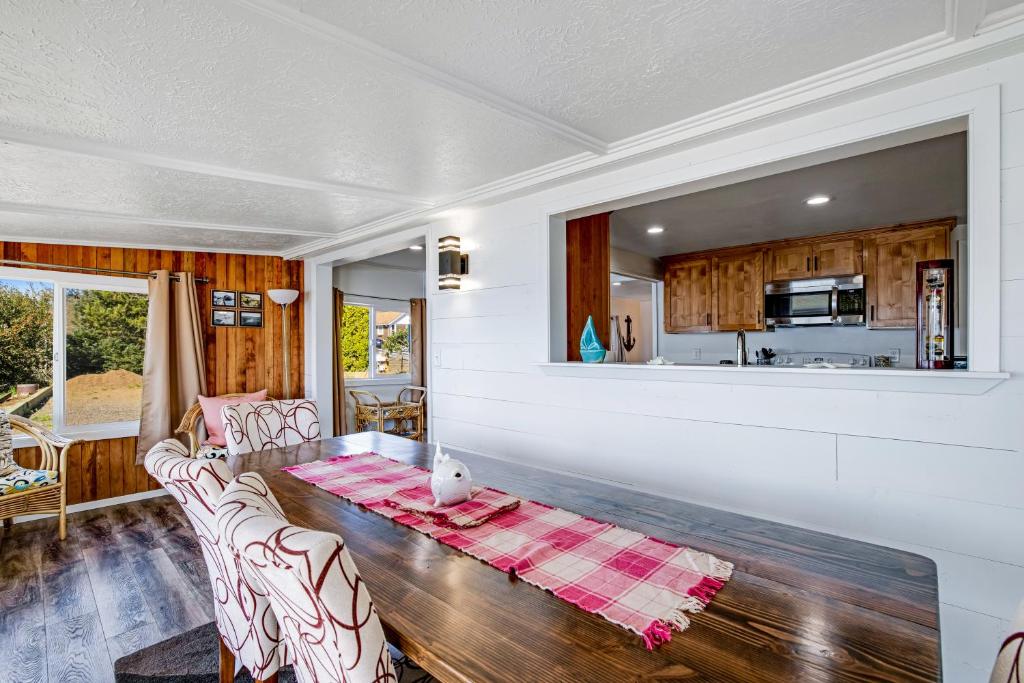In the image, the scene captures the interior of a home, specifically focusing on the dining room area that seamlessly transitions into the kitchen. Central to the dining room is a long, dark wooden table adorned with a red and white checkered table runner. At the center of the runner sits a round, white teapot. Surrounding the table are four white chairs, each featuring distinctive dark red abstract designs. One side of the table is positioned close to a wooden wall, which displays a window offering a glimpse into the kitchen.

The kitchen area visible through the window boasts brown cabinets with a built-in microwave above the stove, alongside a variety of other appliances. The wall also houses a window that looks out to the exterior of the house. The dining room wall, which doubles as an entranceway into the kitchen, helps merge the spaces into one cohesive setting. The shot, depicting a modern setting within a home with hints of classic elements like wood paneling and stucco-textured ceilings, also includes details such as ceiling lights and an anchor decoration hanging in the background.